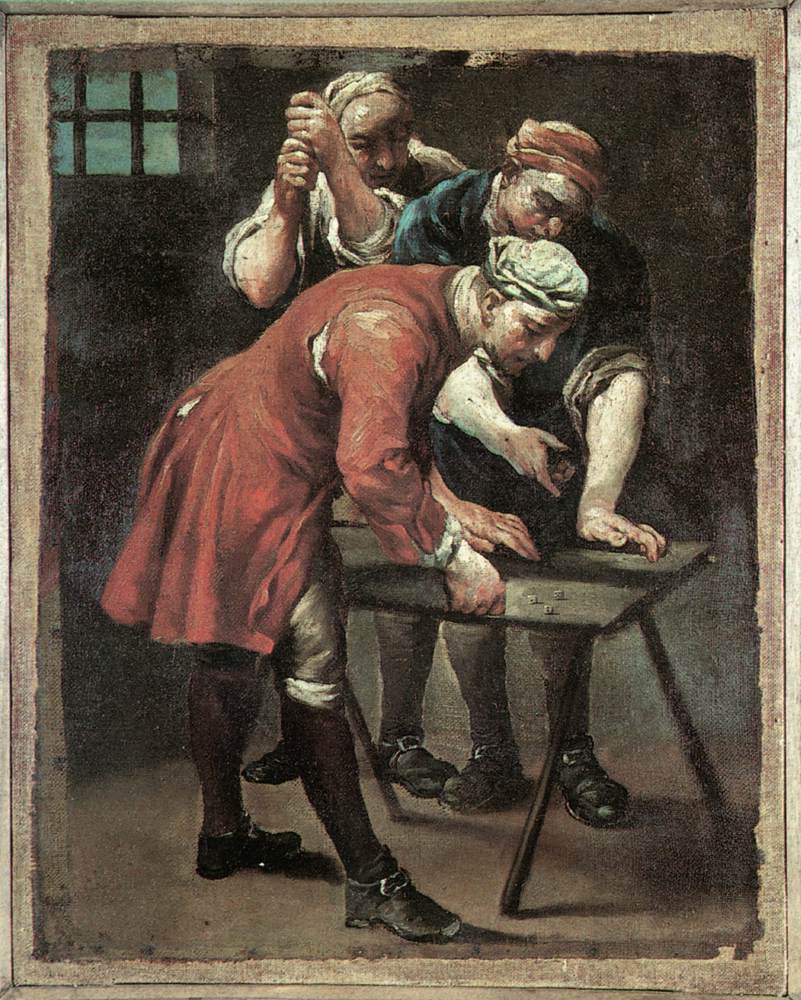This detailed Renaissance-style painting depicts a somber scene involving three men engaged in a tense, quiet moment around a small, angled table with three dice. The man in the foreground, dressed in a torn red coat, white hose, and black shoes with buckles, kneels beside the table, focusing intently on the dice. A white scarf or hat covers his head, adding to his weathered appearance. Opposite him, another man with a reddish headscarf and a blue shirt with rolled-up sleeves leans in, sharing the same intense gaze at the dice. Standing behind them, a third man, dressed in white with rolled-up sleeves, grips a stick with both hands, also peering at the dice. The dimly lit room, accentuated by the dark brown floor and walls, a barred window in the upper left, and an overall dark and moody palette, suggests an oppressive atmosphere, possibly a prison. The painting's edges are irregular and torn, hinting at its age and the story it encapsulates. The figures are depicted with smooth, flowing lines, typical of Renaissance artistry, contributing to the piece's historical authenticity.